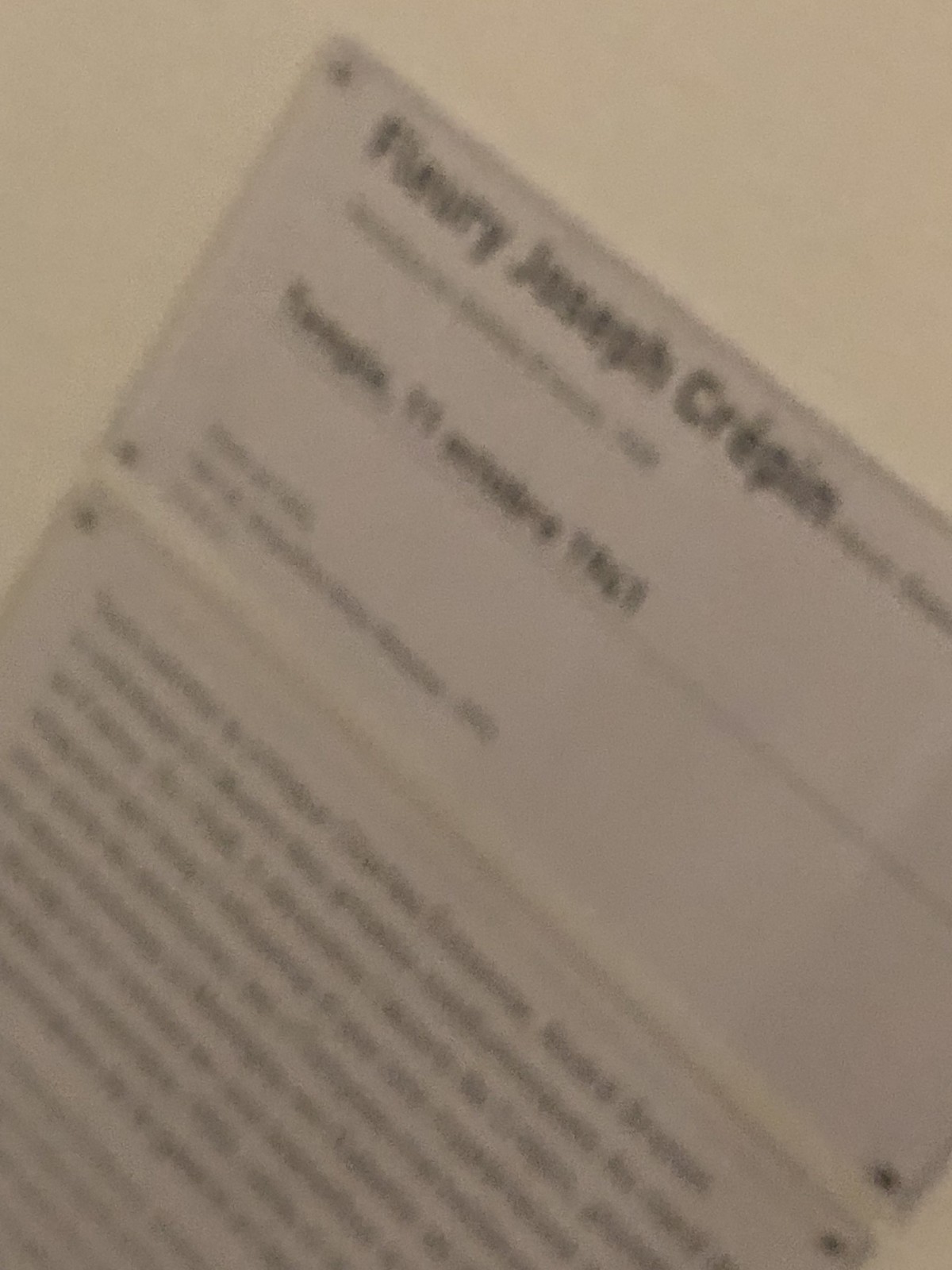This photograph captures a distant and blurry view of a wall adorned with what appear to be plaques or a piece of paper, taken at a steep angle, making the text difficult to discern. The background wall is an off-white cream color, providing a neutral backdrop. The prominent plaque or piece of paper seems to have a name on it. The first name is unclear, possibly starting with an "F." The middle name clearly reads "Joseph." The last name appears to be "Crépin," with an accent mark faintly visible over the "é." Below the name, there seems to be a date or a year, which looks like it might be "1961."